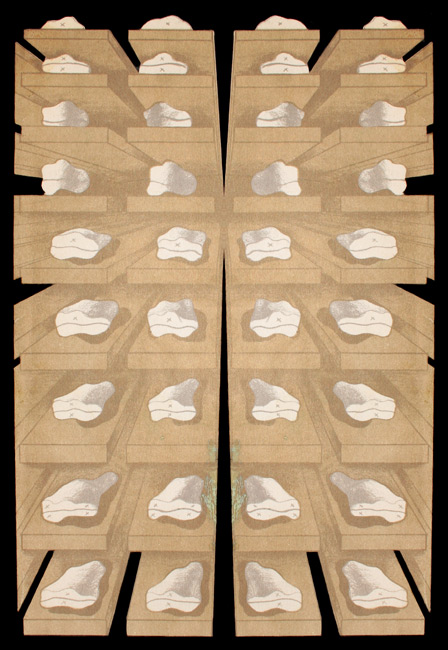This is a highly detailed illustrated drawing by Sorin Dumitrescu, created in 1978 for the cover of Nichita Stănescu's "Epica Magna," rendered in the style of fantastic realism. The image, in portrait orientation, depicts a complex structure of shelves viewed from the side, with the shelves extending horizontally and vertically in a grid-like pattern. There are nine horizontal and four vertical rows, totaling 36 sections, filled with white cloths that resemble towels or sections of bone shaped like pork chops. The primary colors are black, white, light brown, and shades of gray, with a solid black background creating a stark contrast. The intricate shading and shadows around the items enhance the depth and three-dimensionality of the scene, making it appear almost stone-like. The composition is strikingly central, occupying the majority of the frame, which gives the illustration a balanced and cohesive look.